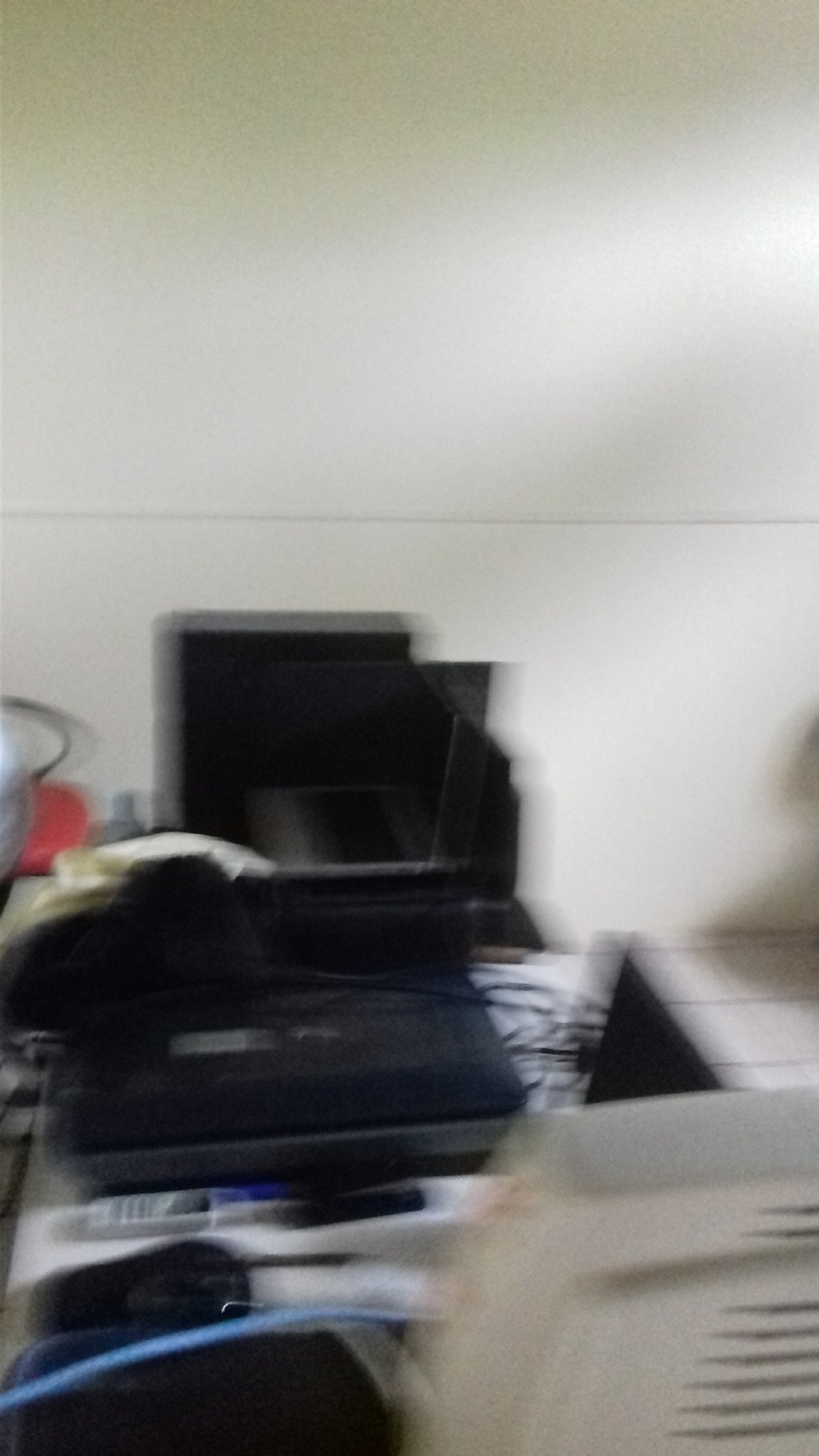The photograph, though blurry and out of focus, depicts a cluttered desk setup within an office or study room. The background features a white wall with a prominent horizontal line running through its center. On the desk below, to the left, there is a gray object, likely a remote control or an old-style cell phone, surrounded by various items. To the right of this gray object is a black, cube-shaped box which may be a gaming console or another electronic device. Prominently, closer to the camera, there is a black briefcase resting atop a white surface. In front of the briefcase, slightly to the left, is a small black object that appears to be a computer mouse. Additionally, a blue cable extends in front of these items, hinting at some connectivity between them. To the right of the mouse, there is a white object with a gray top and multiple black horizontal lines below it, resembling a Wi-Fi router. The varied items on the desk suggest a mix of computer parts and peripheral devices, and despite the image’s lack of clarity, the setting conveys a sense of technological clutter and utility.